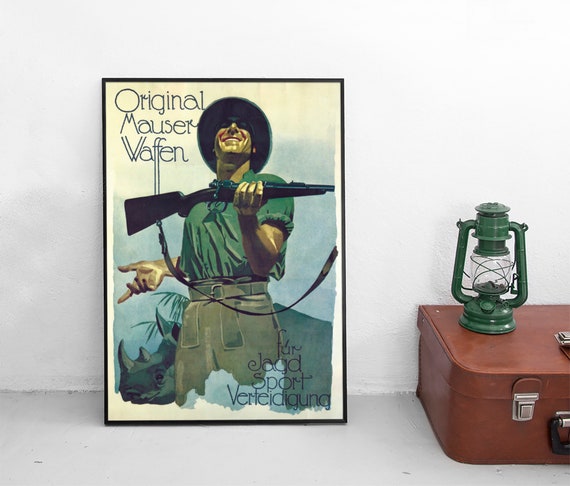This image portrays a rustic and nostalgic scene. In the bottom right-hand corner, there is a brown leather suitcase with stainless steel latches, resting flat on a white floor. On top of the suitcase sits an old green lantern, featuring an iconic design with a glass center, though it lacks a wick. Leaning against a white wall to the left of the suitcase is a poster, enclosed in a narrow black frame, which features a man in safari attire. He wears a safari helmet and has an olive green shirt with rolled-up sleeves, paired with khaki green pants and a mesh belt. The man appears to be Caucasian and is depicted in a cartoon or colored pencil drawing style. He holds a brown rifle with a shoulder strap using his left hand, extending it forward and pointing to the right, while his right hand is bent at the elbow with his palm turned upward. The backdrop of the poster shows a mountain and a blue sky. Text at the top left corner in thin, vintage-style black print reads "Original Mauser Waffen", and additional text at the bottom right says "Jagged Sport Werdengang", likely in German.